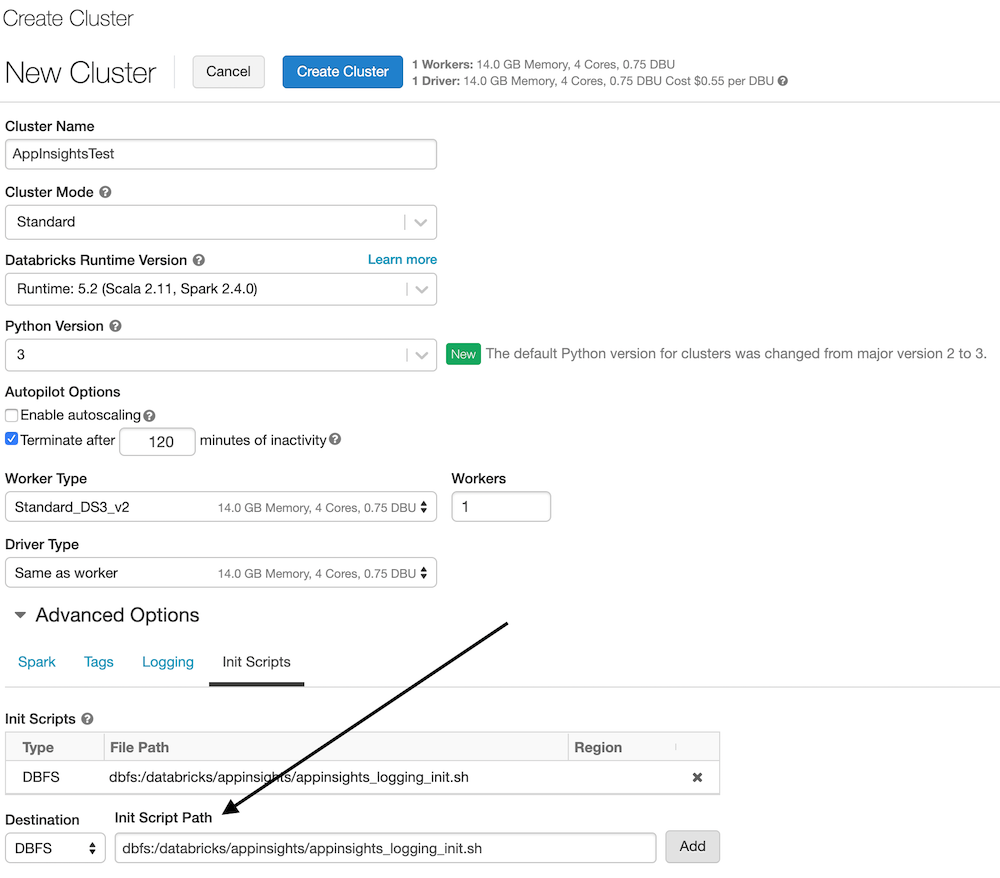In this image, we see a detailed user interface for creating a new cluster. The background is predominantly white. At the top left is the heading "Create Cluster" in black text. Just beneath, there's a subheading "New Cluster." To the right of the subheading, there are two buttons: a gray "Cancel" button and a blue "Create Cluster" button with white text. Adjacent to these buttons is a gray text block detailing resource specifications, which reads: "One worker, 14 GB memory, 4 cores, 0.75 dBu. One driver, 14 GB memory, 4 cores, 0.75 dBu, costs $0.55 per dBu."

Below these elements, there is an extensive section with multiple fields and drop-down menus intended for cluster configuration, with labels such as "Cluster Name," "Cluster Mode," "Databricks Runtime Version," "Python Version," "Autopilot Options," "Enable Autoscaling," "Terminate After Minutes of Inactivity," "Worker Types," "Workers," and "Driver Type."

Further down, an expandable section is marked with a down arrow labeled "Advanced Options," revealing four selectable tabs: "Sporks," "Tags," "Logging," and "Init Scripts." The "Sporks," "Tags," and "Logging" tabs are highlighted in blue text, whereas the "Init Scripts" tab is selected, indicated by a black underline.

Within the "Init Scripts" section, there are fields for specifying script details including a "Destination" drop-down menu and an "Init Script Path" text field. There’s a text field along with an "Add" button at the bottom right, colored gray. Additionally, there is a black arrow drawn that points to the "Init Script Path" text field.